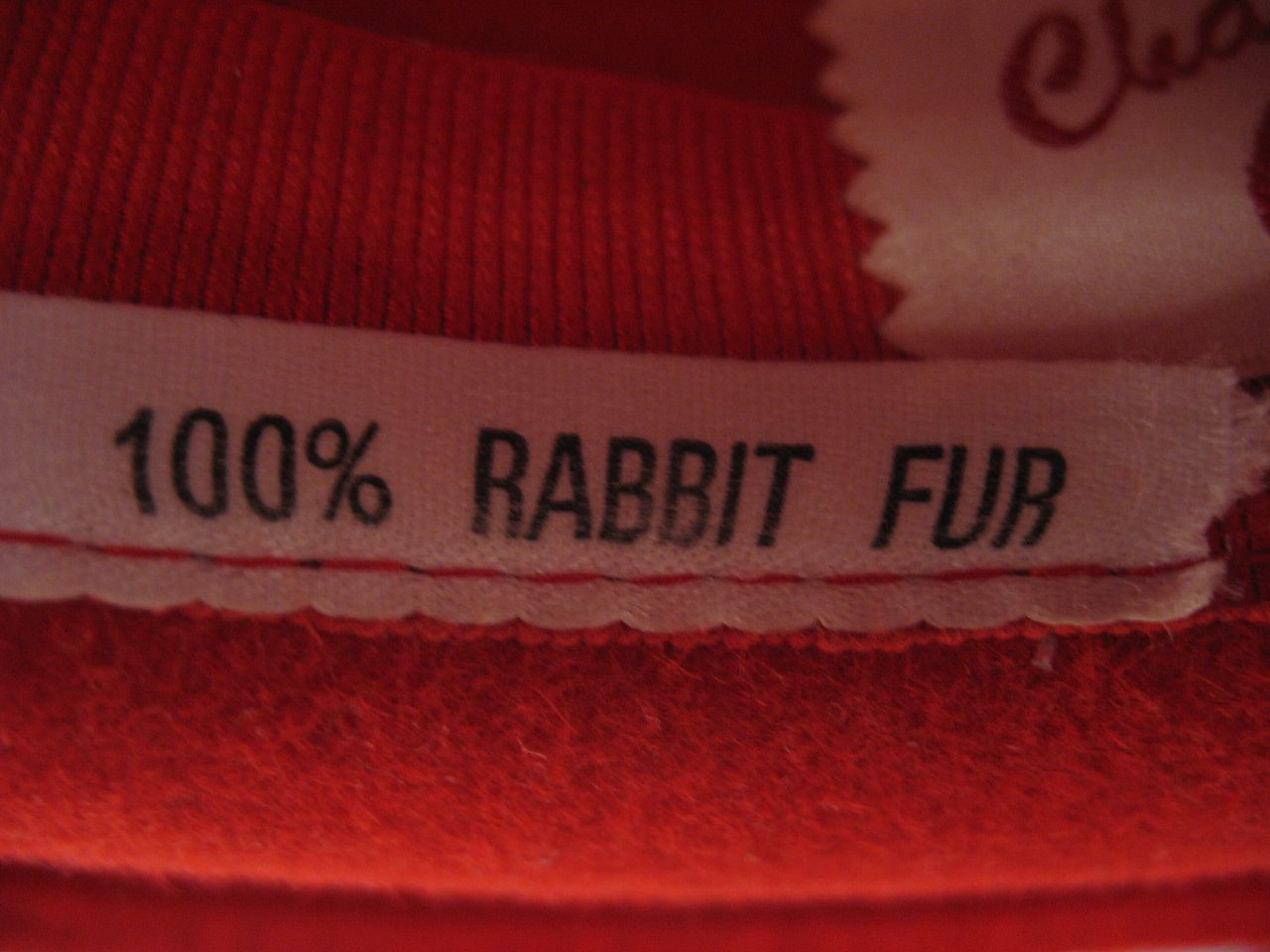A close-up photograph captures a white cloth tag meticulously sewn onto a piece of vibrant red clothing. The rich red stitches securing the tag are prominently visible, adding a touch of contrast to the composition. Edges of the white tag slightly extend beyond the stitching, contributing to its prominence in the frame. In the center of the tag, elegant black lettering reads "100% rabbit fur," indicating the luxurious material of the garment. The intricate details in the image accentuate the craftsmanship and quality of the fabric.